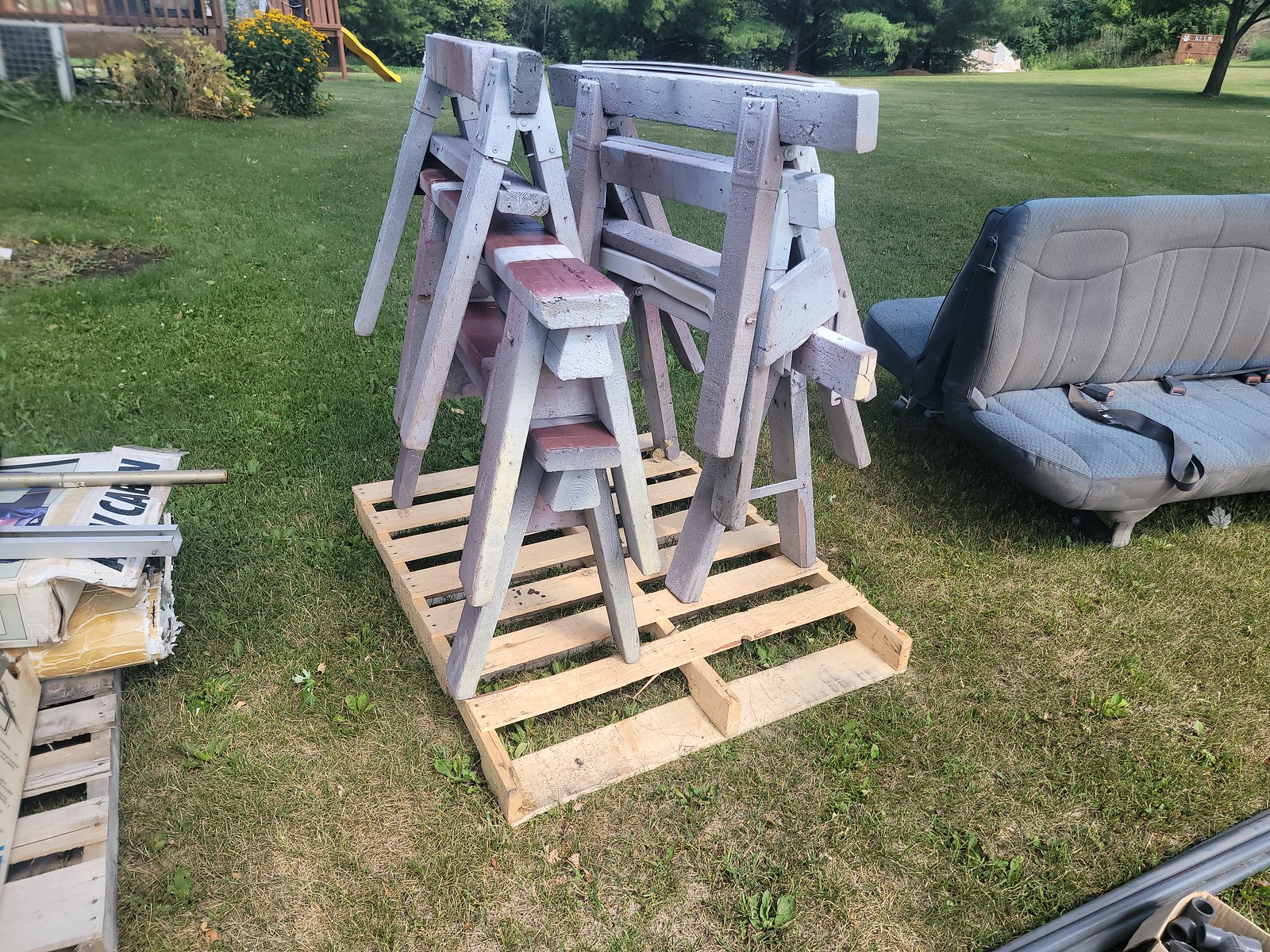The image depicts a suburban lawn with a mix of green and brown grass, featuring patches where dirt is visible. Dominating the foreground are two old car bench seats set back-to-back with visible seatbelts, suggesting they were removed from a larger vehicle, possibly a van. Adjacent to the seats, there is a light-colored wooden pallet, on which six gray saw horses are arranged in two side-by-side stacks, each with three on top of one another. Another wooden pallet with obscured gear is positioned to the left, while metallic tubes or poles lie on the grass at the bottom edge of the frame. In the background, a children's playground set with a yellow slide and a brown tree trunk is visible, suggesting the scene is likely a yard sale at a suburban home. A partial view of a wooden deck, several plants including one with yellow flowers, and a tree line complete the background scenery.